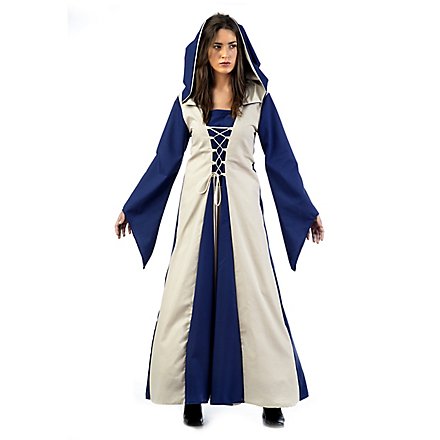The image features a young woman, likely in her 20s, with long brown hair cascading to her shoulders. She is standing against a stark white background, looking off to the right with pursed lips. Her attire is a detailed costume that includes a long, flowing blue and white dress. The outfit consists of a white vest-like upper portion that ties in the middle and extends to her ankles. A significant part of her ensemble is a blue cape-like garment with a hood draped over her head. The sleeves of this cape are royal blue, large, and extend well past her wrists, creating a dramatic, flowy effect. Down the center of her costume is an additional royal blue section, complemented by lace-up detailing. She completes her look with black shoes. The way she stands with her arms somewhat out to her sides suggests she is modeling the costume, which appears intricate and suited for an event like Halloween rather than everyday wear.